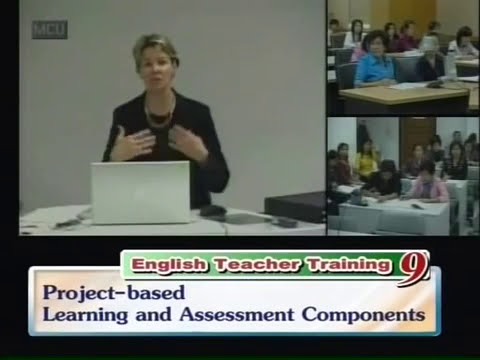In this Zoom or conference call image, titled "English Teacher Training: Nine Project-Based Learning and Assessment Components," we see a split-screen layout with three distinctly different sections. In the prominent top-left section, a Caucasian woman with short blonde hair is standing behind an all-white desk, wearing a black shirt paired with a pearl or gold necklace, and stationed in front of a silver laptop. Papers are scattered around her desk, indicative of active engagement. The label "MCU" appears in the top left corner of this section, possibly signifying a logo or identifier. To the right, the screen is divided into two smaller images. The upper right shows several students sitting at light plywood-colored desks, while the lower right section showcases predominantly Asian students seated at white desks, suggesting two different classroom settings connected through the video feed. Below these visual elements, a green banner with red text reads: “English Teacher Training: Nine Project-Based Learning and Assessment Components,” emphasizing the educational focus of the call.